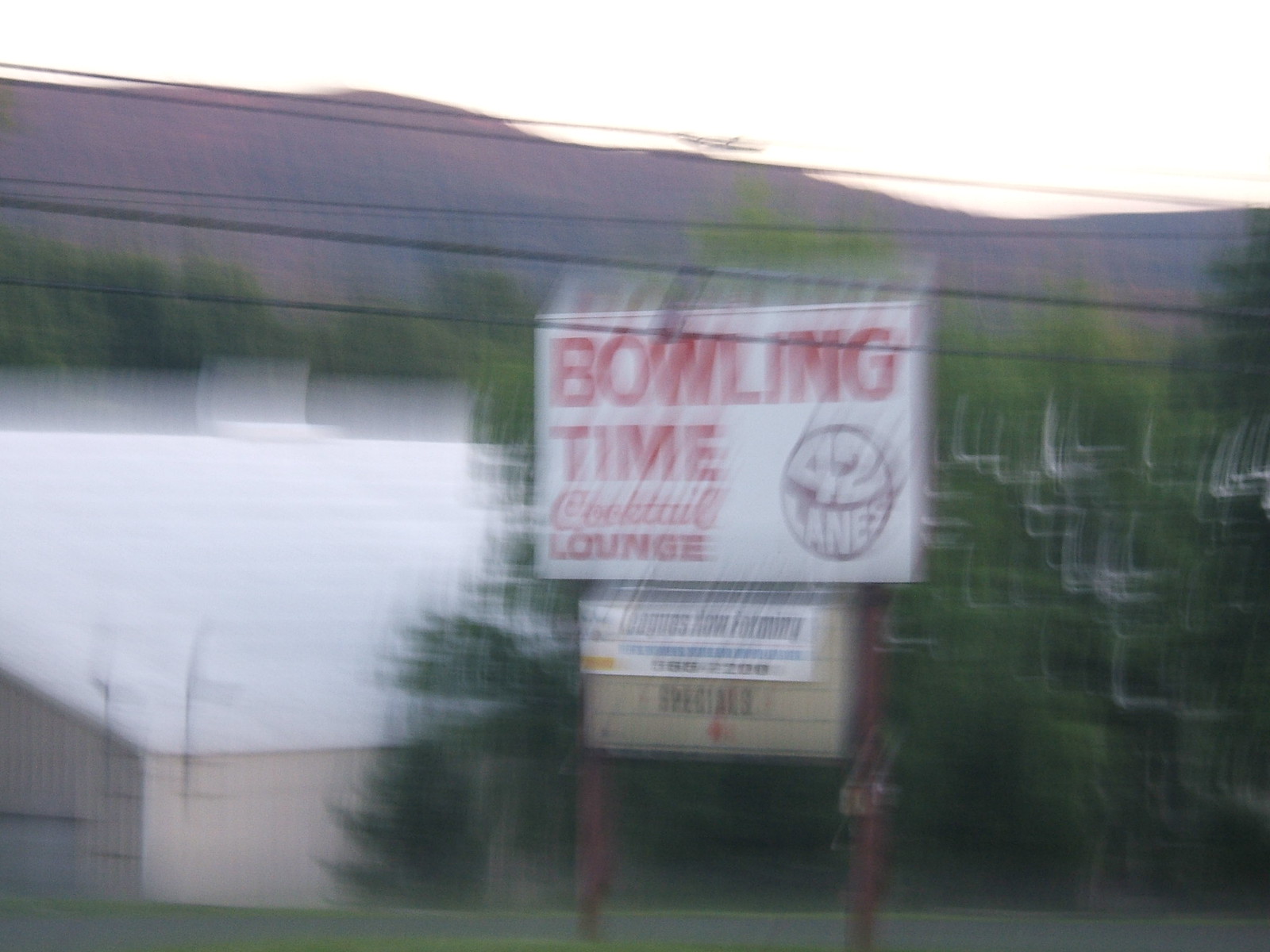The image features a large tan building with a brilliant white roof, nestled in a scenic background of trees, hills, and a setting sun. Stretching across the horizon are electrical or telephone lines. In the foreground, there's a prominent sign standing on two wooden poles. Despite the image's overall blurriness, the sign is legible: it reads "Bowling Time" and "Cocktail Lounge" in red letters on a white background, featuring an illustration of a bowling ball with "42 lanes" written across it. Below this, there's a moveable letter sign partially covered by a white banner with black text that announces "Leagues Now Forming," accompanied by an unreadable phone number and some green text. Surrounding the sign is some greenery, adding to the depth and detail of the scene.